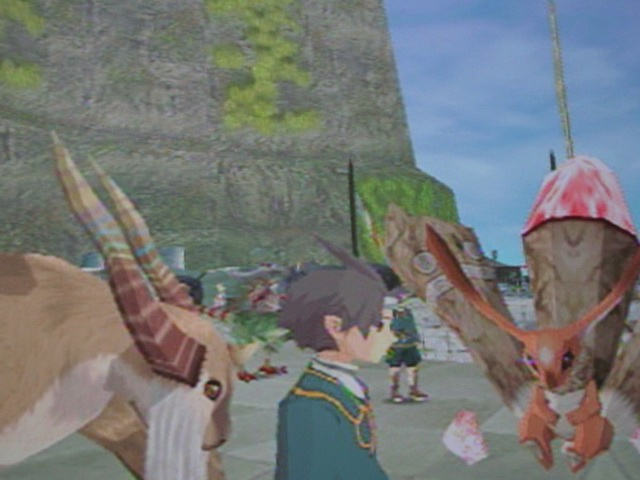In this motion capture still from a computer game, a whimsical scene unfolds in front of a partially visible, pyramid-shaped building made of gray stone and covered with mottled green patches of moss. Various cartoonish figures are milling around, adding life to the setting. At the forefront stands a humanoid character with an elf-like appearance, featuring pointed ears and shown in profile with their left side facing the viewer. This character is dressed in a green jacket, exuding a simplistic yet charming design. Behind this character looms a large, ox-like creature, distinguished by its brown coat, white whiskers, and long, spiraling, striped horns. Completing the scene, a rabbit sits in front of the humanoid character, gazing directly toward the viewer, grounding the image with a touch of curiosity.